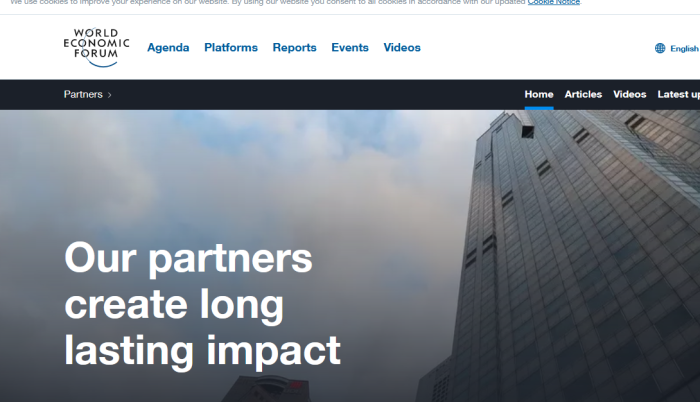The image depicts a webpage from the World Economic Forum's website. In the top left corner of the image, "World Economic Forum" is prominently displayed. To the right of this title, a navigation menu includes categories such as Agenda, Platforms, Reports, Events, and Videos. On the far right of this menu, the word "English" is accompanied by a globe icon, indicating language selection options.

Beneath the "World Economic Forum" title, the word "Partners" appears with an arrow pointing to the right. Adjacent to this, on the far right side of the image, another set of categories is visible: Home, Articles, Videos, and Latest. Each category is presented in white text.

The central background of the image features a large building on the right side. The building appears to have several windows that are either missing or blacked out. To the left of the building, the sky is visible and filled with clouds.

At the bottom left of the image, overlaying the picture, text reads: "Our partners create long-lasting impact." Additionally, at the very top of the image, partially visible, is a notice about cookies which states: "We use cookies to improve your experience on our website. By using our website, you consent to cookies in accordance with our updated cookie notice." The phrase "cookie notice" is highlighted in blue text with an underline.